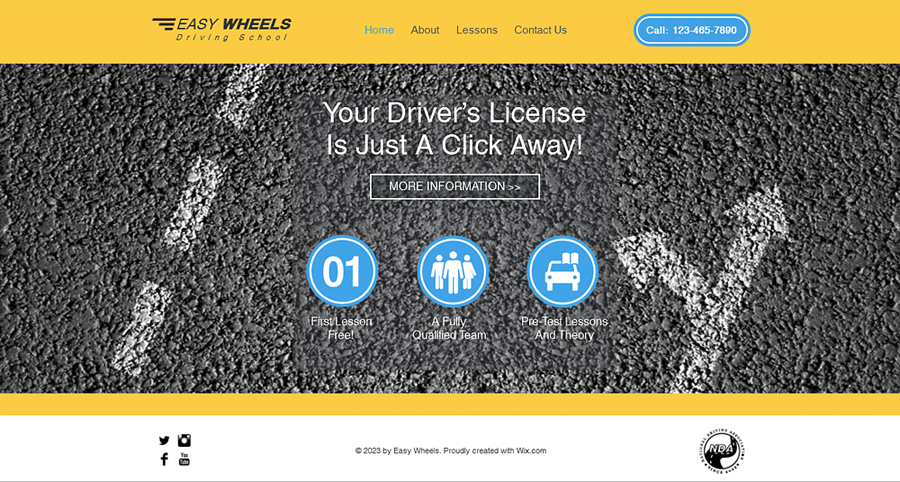The image displays the homepage of the Easy Wheels driving school's website. The top portion features a yellow background with a yellow bar stretching across the top and a thinner yellow bar at the bottom. Central to the image is an asphalt road with white lines. In the top-left corner, the Easy Wheels logo and text are visible, indicating "driving school." To the right of the logo, a navigation menu with tabs labeled "Home," "About," "Lessons," and "Contact Us" is present. Adjacent to these tabs is a blue button or bubble with a phone number, labeled "Call Us."

Below the main navigation, white text reads, "Your driver's license is just a click away." Directly underneath this message, there is a white button outlined in a white box labeled "More Information." Lower on the page, three blue bubbles contain additional information, stating "First Lesson Free," "Qualified Team," and "Pro Lessons."